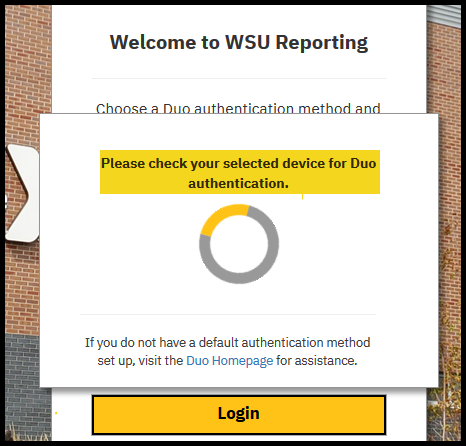This image is a cropped and edited screenshot of a section of a website displaying a Duo authentication prompt for WSU reporting. At the top of the image, on a white background, the text reads, "Welcome to WSU Reporting." Below this, it says, "Choose a Duo authentication method."

Taking up the center of the page is a large white square overlay box. Within this box, at the top, there is a prominent large yellow box with the message, "Please check your selected device for Duo authentication." 

Further down in this overlay box, there is a circular icon with a yellow segment on the top left. Just below this icon, a message advises, "If you do not have a default authentication method set up, visit the Duo homepage for assistance," with "Duo homepage" hyperlinked in blue text.

At the bottom of the white overlay box, a large yellow login button is visible. This button is outlined in black, and the word "Login" is centered in bold black letters.

In the background of the entire image, a photo of a brick building is faintly visible, with bricks peeking through on the left and right edges. There is also a partial view of a white 'X' sign on a building, adding to the urban context of the scene.